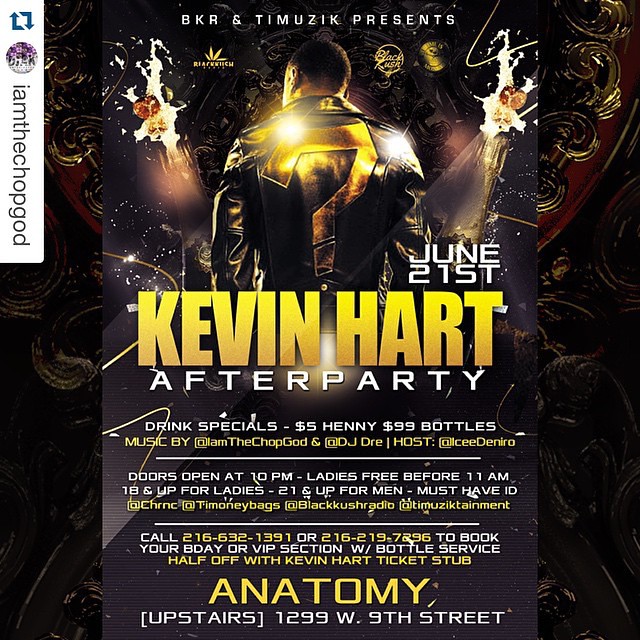This promotional poster, designed with a striking black and gold theme, announces an exclusive Kevin Hart After Party presented by BKR and Timusic on June 21st. Dominating the central area, the name "Kevin Hart" is boldly highlighted in vibrant yellow-gold lettering. The poster features an image of a person wearing a black leather jacket adorned with a golden question mark and artistic white paint splatters, facing away from the viewer against a dark, ornate patterned background.

Event details include drink specials: $5 Henny and $99 bottles, with doors opening at 10 PM. Ladies enter for free before 11 AM, with the event open to women 18+ and men 21+. VIP sections and birthday bookings, complete with bottle service, are available at a 50% discount for those with a Kevin Hart ticket stub. To reserve, attendees are prompted to call 216-632-1391 or 216-219-7296. The venue, Anatomy, is located upstairs at 1299 West 9th Street. Additional promotions feature Instagram handles @iamthechopgod, @djdre, and host @iciedeniro.